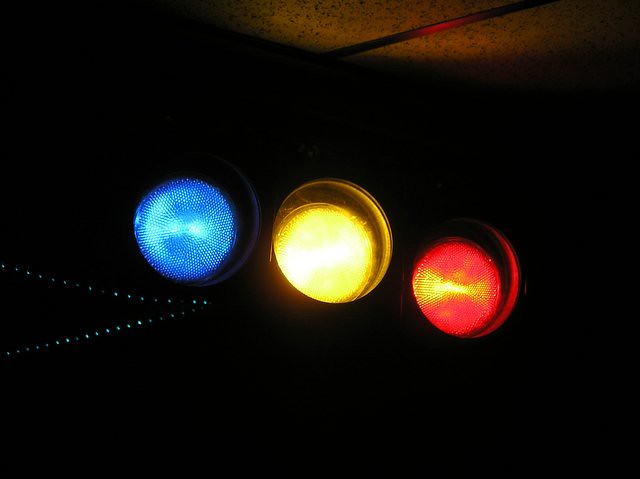The image captures a dark room illuminated only by lights resembling a horizontally-aligned traffic light fixture, with three bulbs: blue on the left, yellow in the center, and red on the right. These bulbs cast a faint glow onto the ceiling, which is a tiled, push-up variety typical of office buildings. Below the traffic lights, a delicate string of white-blue fairy lights hangs on the lower left side of the image, forming a V-shape. The entire scene is shrouded in darkness, with no other visible elements, giving a sparse and enigmatic atmosphere.